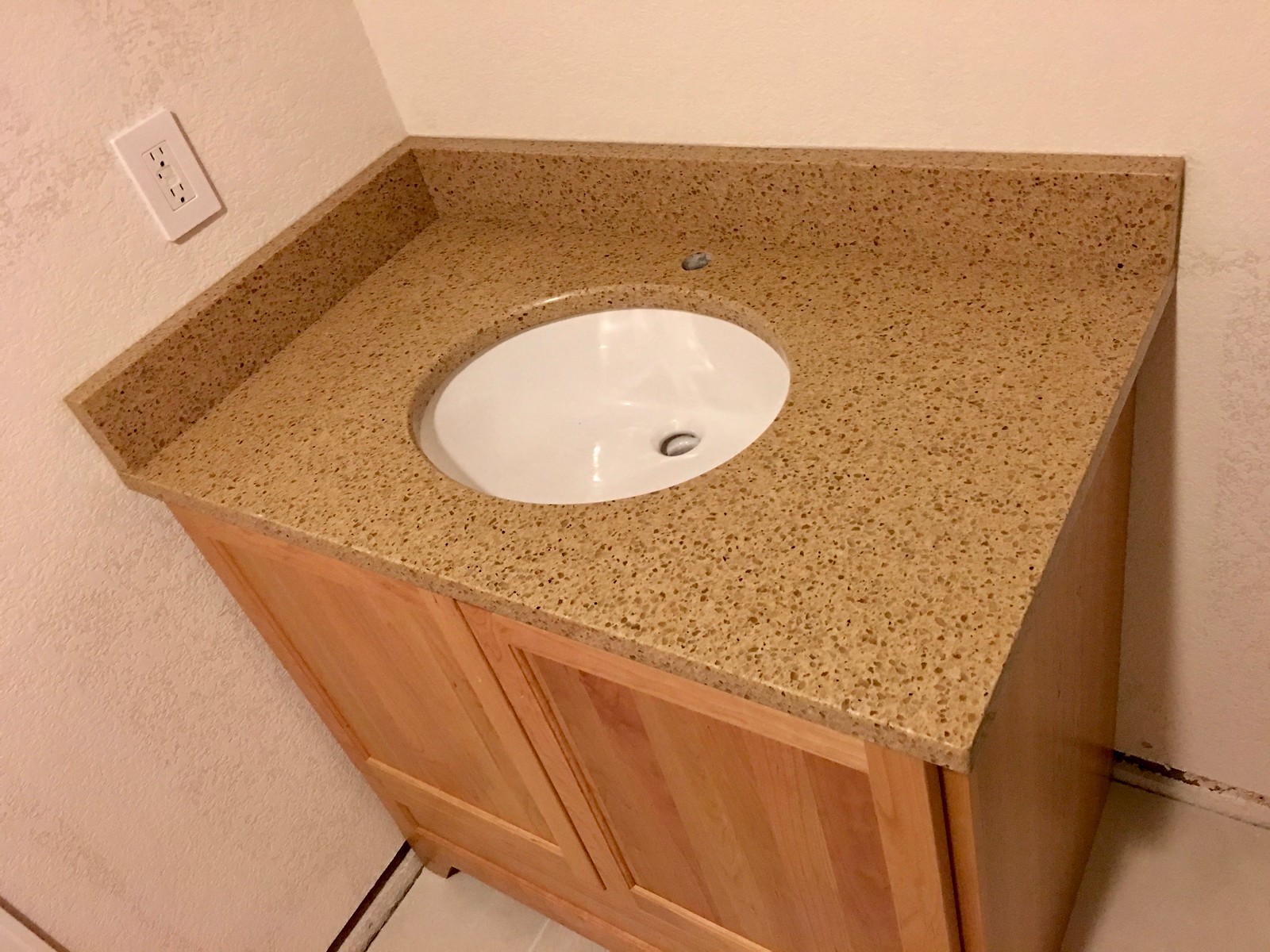The image depicts an unfinished bathroom basin situated in a corner of a room. The scene appears to be a bathroom, though no other typical bathroom fixtures are visible. The walls are painted white, contributing to a stark, minimalist appearance. 

On the left wall, there is a dual plug socket, indicating potential for electrical appliances to be used in the area. The basin itself is placed snugly against the corner, with a noticeable offset in the photograph composition, creating irregular angles.

The basin is crafted from a brown, somewhat unsightly material, possibly marble or Corian, and features a built-in splash guard on both the side and back. Centrally located within the basin is a white sink made of either ceramic or porcelain, which includes a drain hole currently lacking a cover. 

Additionally, there is a secondary hole behind the sink, presumably designed for a fixture, though it remains uninstalled. Supporting the basin is a pale wooden cabinet featuring two outward-opening doors. The floor beneath the setup is covered in gray, square tiles, adding to the room's unfinished yet functional aesthetic.